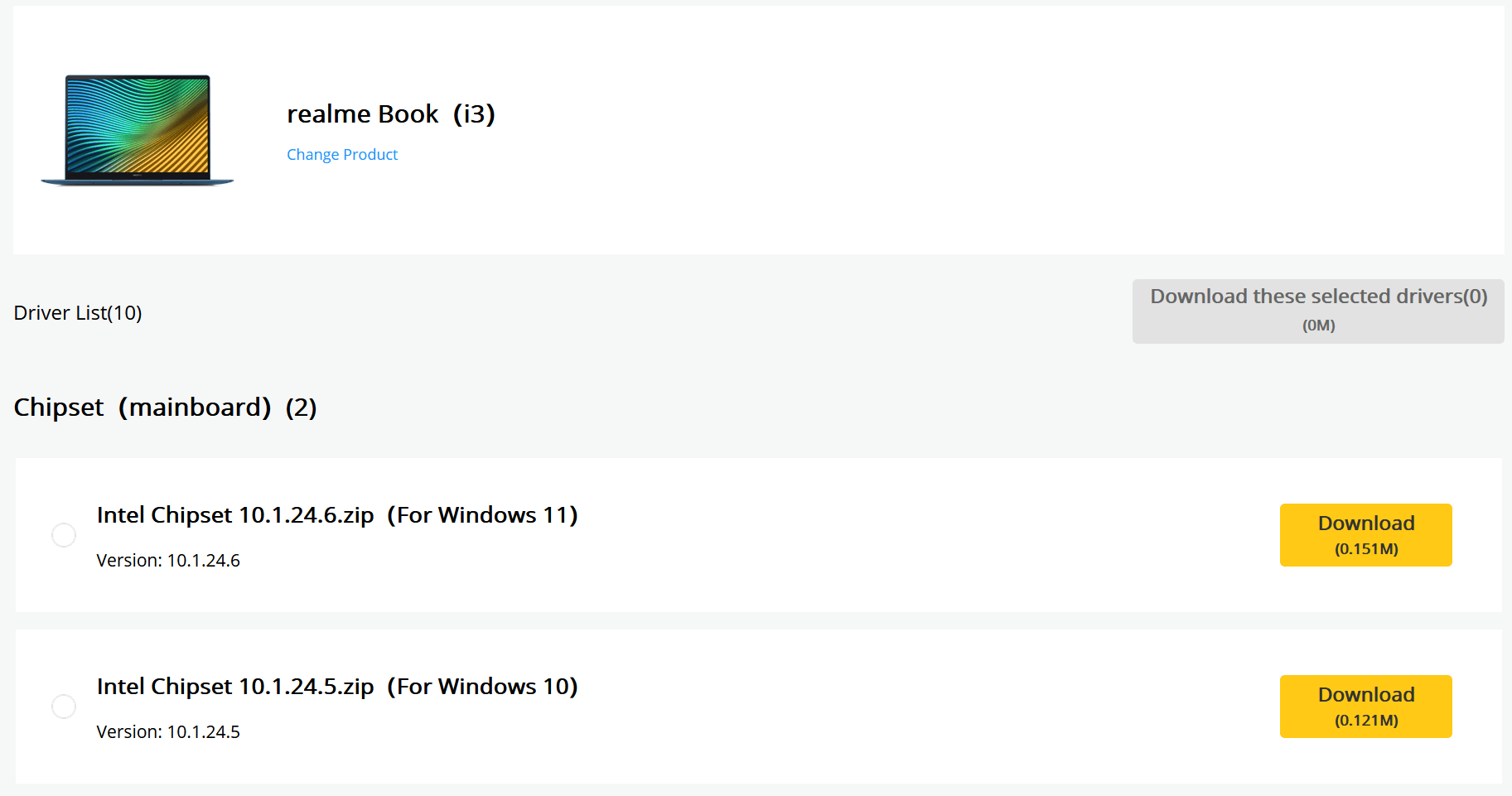**Detailed Caption for Image:**

The image showcases a laptop, specifically identified as a Realme Book (i3), with a sleek design that resembles a MacBook Pro. The laptop is open, revealing its screen which displays a distinctive pattern of half-barred black lines with swirling blue, green, and yellow colors. Below the laptop's brand name, there is blue text labeled "Change Product".

On the screen, a smaller text area is visible, labeled "Driver List," indicating that the laptop is displaying a list of drivers available for download. There are ten options listed under various categories. At the far right, a gray button with the text "Download the Selected Drivers" is present, indicating functionality for driver selection and download. Below this button, there is a notation of "0.0M" in brackets, likely describing the zero megabytes selected for download so far.

Under the "Chipset" category, which includes a sub-heading in parentheses "(Main Board) (2)", there are two driver options:

1. **Intel Chipset 10.1.24.6.zip for Windows 11**: This is for version 10.1.24.6, downloadable at a size of 0.151 MB.
2. **Intel Chipset 10.1.24.5.zip for Windows 10**: This is for version 10.1.24.5, downloadable at a smaller size of 0.121 MB.

Each driver option has a corresponding yellow download button on its right side. The overall background of the screen is white, creating a clean and spacious appearance.